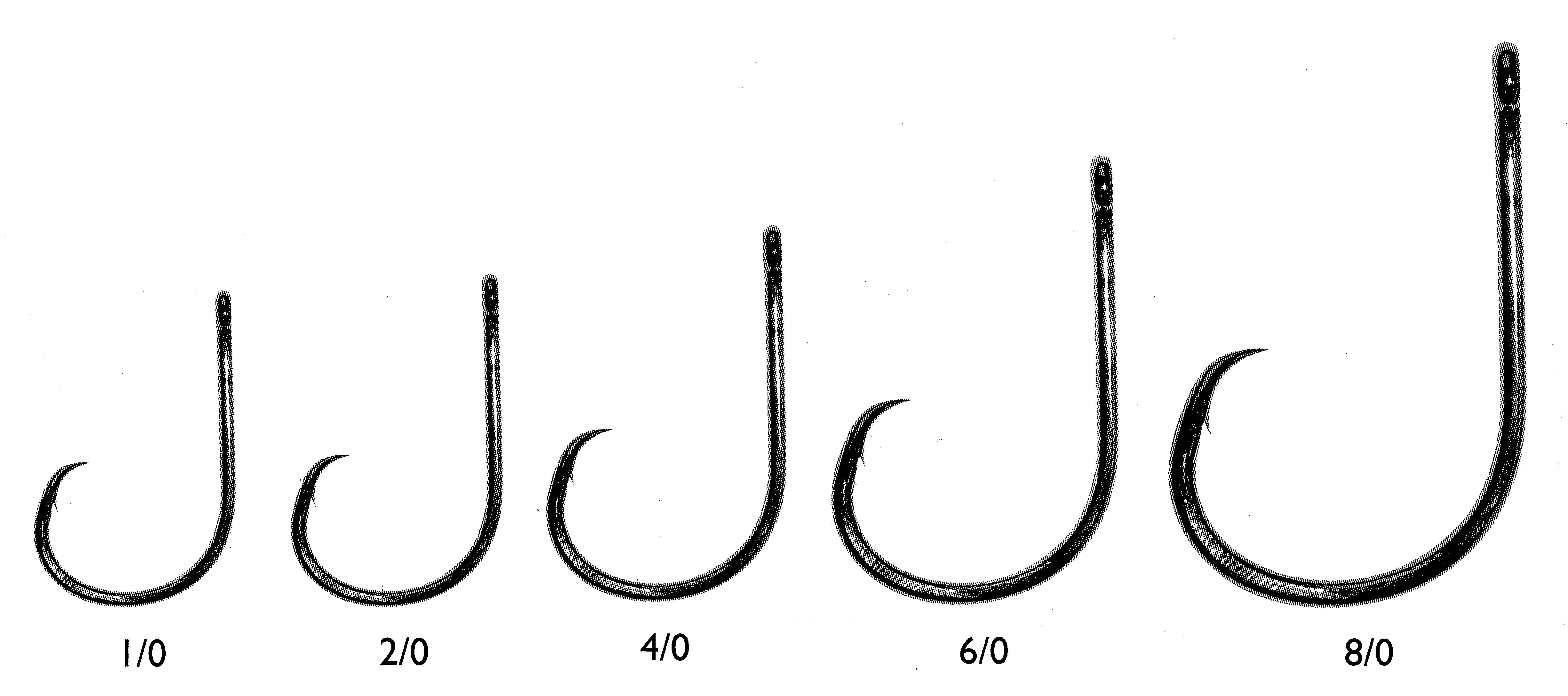The image depicts a set of five metal fish hooks arranged in a horizontal row on a white background. Each hook, made of a blackish-silver metal, increases in size from left to right. The smallest hook on the far left is marked with "1/0," followed by "2/0," "4/0," "6/0," and the largest on the far right marked with "8/0." All hooks share a similar design, starting with an eyelet at the top and curving downward in a J shape, ending in a sharp point. Additionally, each hook features a small barb near the point to help secure the catch. The contrasting colors make the details, including the numbers and barbs, clearly visible against the white background.